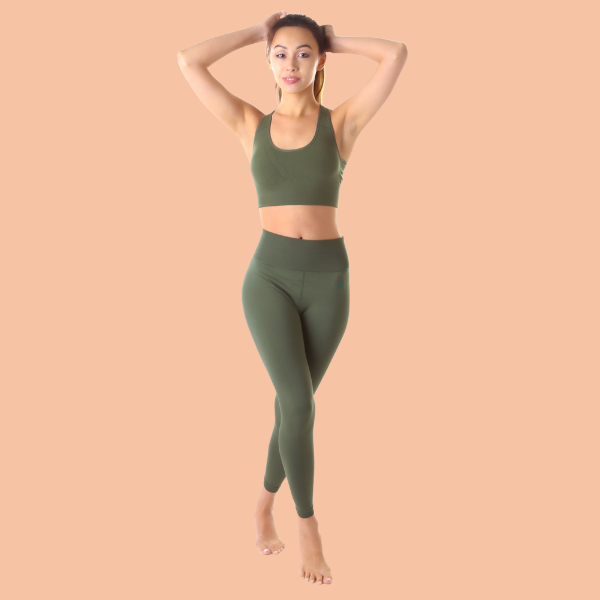In this image, a young woman stands gracefully in a featureless peach-colored space, likely a studio setting. She is posing in an olive green workout outfit consisting of a matching sports bra and high-waisted yoga pants, which reveal part of her belly and belly button. Her fair skin and dark brown hair, tied back in a ponytail, frame her face as she looks directly into the camera with a slight smile. Her feet are crossed, one foot positioned on her toes with white nail polish, giving the impression of either a yoga pose or a dance move. The woman appears to be in her early 20s, with a fit and toned physique, suggesting that she exercises frequently. She holds her hands behind her head, elbows out, adding a sense of elegance and strength to her pose.